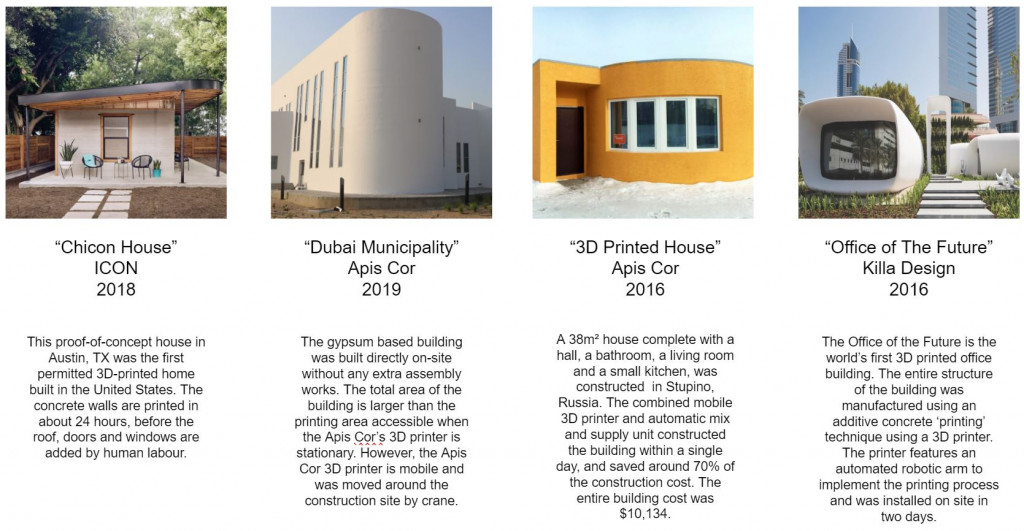The image presents a catalog-like compilation of four futuristic, proof-of-concept house designs, displayed in a landscape orientation with square photographs positioned side by side horizontally. Each photograph has corresponding black text above and below, providing detailed descriptions. 

Starting from the left, the first design, labeled "Chicon House, Icon 2018," is a single-story, flat-roofed, white building situated in an outdoor setting in Texas. It was 3D printed and features a window, patio chairs, and concrete pavers leading up to the entrance, framed by two columns of four rows each.

To the right is the "Dubai Municipality, Apis Core 2019," a smooth, white, multi-story 3D printed building. It has distinctive long rectangular windows spaced vertically along its façade, constructed on-site with a gypsum-based material using an Apis Core 3D printer.

Next is the "3D Printed House," a single-story, flat-roofed structure with a striking yellow-orange color. It includes four rectangular windows and a brown door. Notably, it was built at a remarkably low cost of $10,000.

On the far right is the "Office of the Future, Killa Design 2016," displaying a white, modular, cube-shaped design with curved edges, characterized by large windows. The structure appears elliptical with a recessed entrance and is set against a backdrop of skyscrapers.

The detailed photographic representation combined with graphic design and text underlines the innovative and experimental nature of these 3D printed structures.